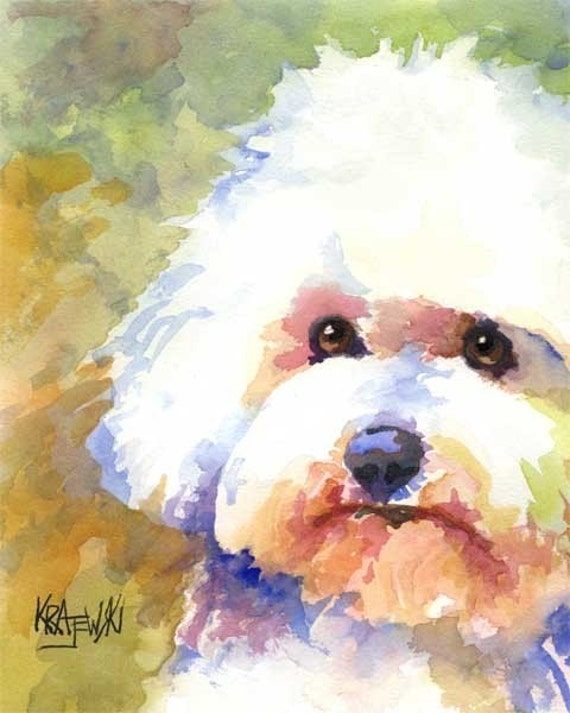This watercolor painting, measuring approximately five inches high by four inches wide, features a detailed portrayal of a fluffy white dog, likely a toy poodle or a small Maltese. The dog's head and upper chest dominate the composition, starting from the lower right corner and extending upward and leftward. The fur is predominantly white, with subtle accents of pink, orange, yellowish-green, and purple lending depth and dimension, especially around the eyes, ears, and mouth. It has expressive brown eyes with black pupils, a black nose, and a downturned mouth. The background transitions from tones of green at the top to yellows and golds towards the bottom left. The painting is signed in the lower left corner with a black cursive signature, reading "KRAEWKI."